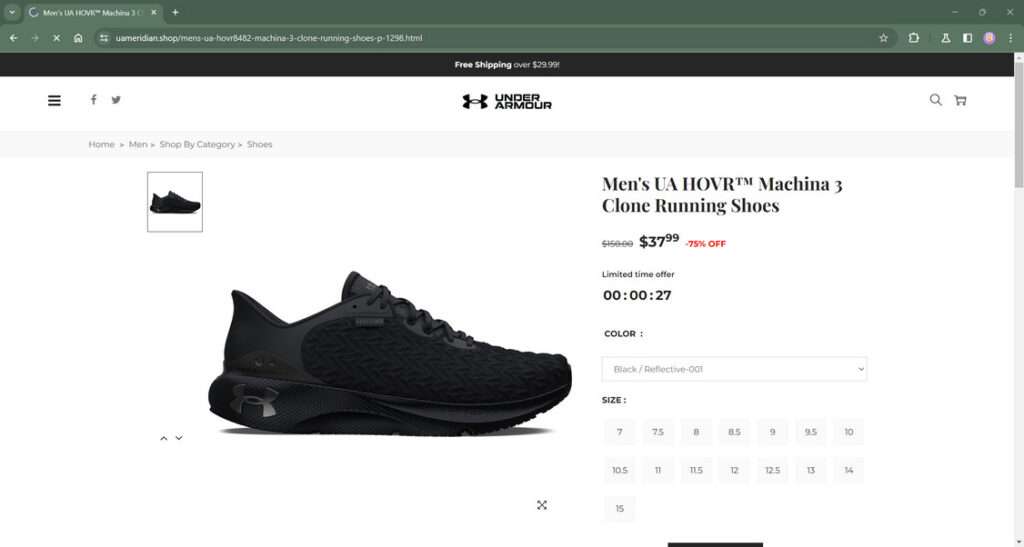Screenshot of a website for selling shoes featuring Under Armour's UA Hovr™ Machina 3 Clone Running Shoes:

- **Top Left Corner**: A navigation tab labeled "Men's UA Hovr Machina 3 Clone," partially cut off. The URL displayed is "american.shop/mens-US-Hovr-8482-Machine-3-Done-Running-Shoes-P-1298.HTML."
- **Left Sidebar**: Three horizontal lines icon in a light gray bezel, along with icons for Facebook and X (formerly known as Twitter).
- **Center**:
  - **Logo**: Under Armour's logo, resembling two "U"s merged together in dark black, followed by the text "Under Armour."
  - **Top Banner**: Black bezel with "FREE SHIPPING" written in bold white text, followed by "over $29.99!" in gray.
- **Main Content**:
  - **Shoe Image**: Displaying a black running shoe.
  - **Size Options**: Sizes listed from 7 to 15, including half sizes.
  - **Product Title**: "Men's UA Hovr™ Machina 3 Clone Running Shoes" in bold text.
  - **Pricing**: Original price "$150" struck through, with the discounted price "$37.99" in black and "75% OFF" in red.
  - **Offer Details**: "Limited Time Offer" in gray, with a countdown showing "27 seconds left."
  - **Color Selection**: Labeled "Color," with black/reflective (001) selected.

The screenshot provides a comprehensive overview of the product page, including detailed pricing, size availability, and design elements.